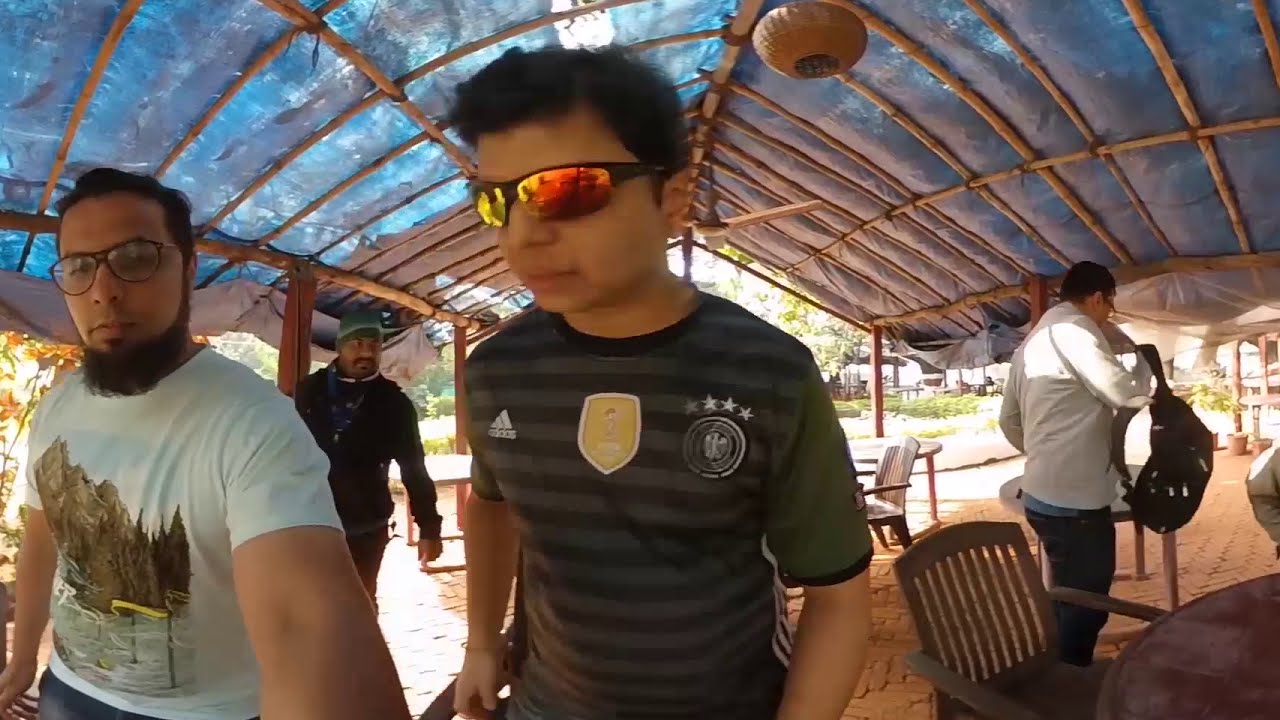The photograph captures a daytime outdoor public gathering beneath a home-built canopy made of sticks covered by a blue tarp. Four men are positioned centrally under the tent, which sits above their heads. The man at the center stands out in a black and gray striped t-shirt featuring star and shield designs, sporting sunglasses with reflective orange and yellow lenses. To his left, a bearded man in glasses wears a white t-shirt adorned with a mountain and lake design. Between them is a man in a black shirt and a greenish-blue baseball cap. The fourth man, with his back turned, wears a white jacket and carries a bag. Surrounding them are wooden tables and chairs, with other people walking around in the background. Lush green trees indicate a summertime setting, and there are no visible text elements in the image. The colors present include light blue, brown, tan, green, and various shades of clothing.